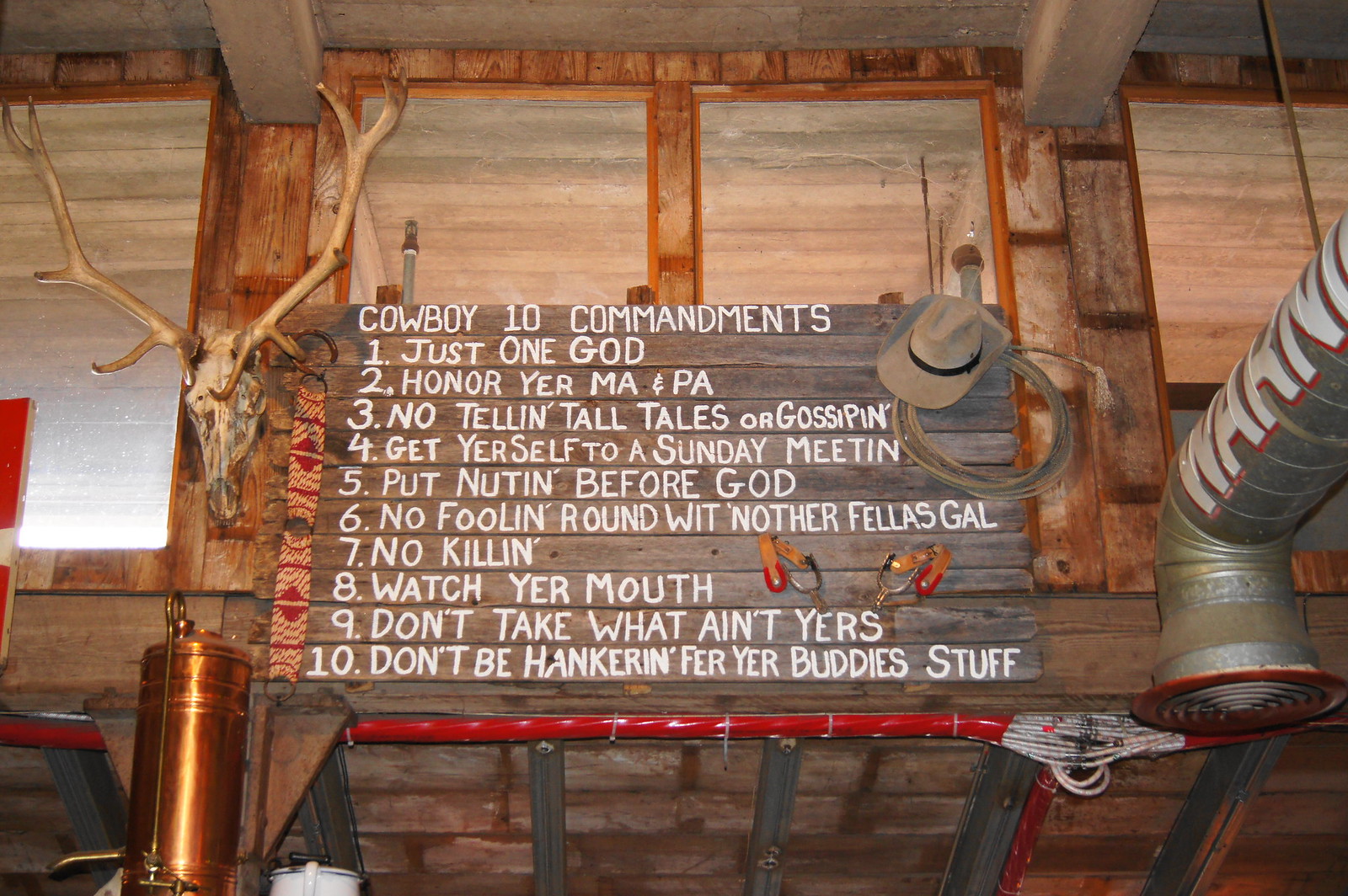The image captures the rustic interior of what appears to be a cowboy-themed bar or café, established within a log cabin. Dominating the center of the image is a large wooden slab with white chalk text outlining the "Cowboy Ten Commandments," which include directives such as "Just one God," "Honor your ma and pa," "No telling tall tales or gossiping," and "Get yourself to a Sunday meeting." The commandments are listed in a straightforward, rustic style. The sign is complemented by various western-themed decorations, including a deer's antler mount on the left, and at the top-right corner of the slab, a cowboy hat and whip are prominently displayed. Accompanying these items are exposed industrial pipes and venting, adding to the rugged ambiance. The color palette is dominated by shades of brown, white, bronze, red, and black, consistent with the wooden interior and vintage décor. This cozy, themed setting creates a charming, historical atmosphere.